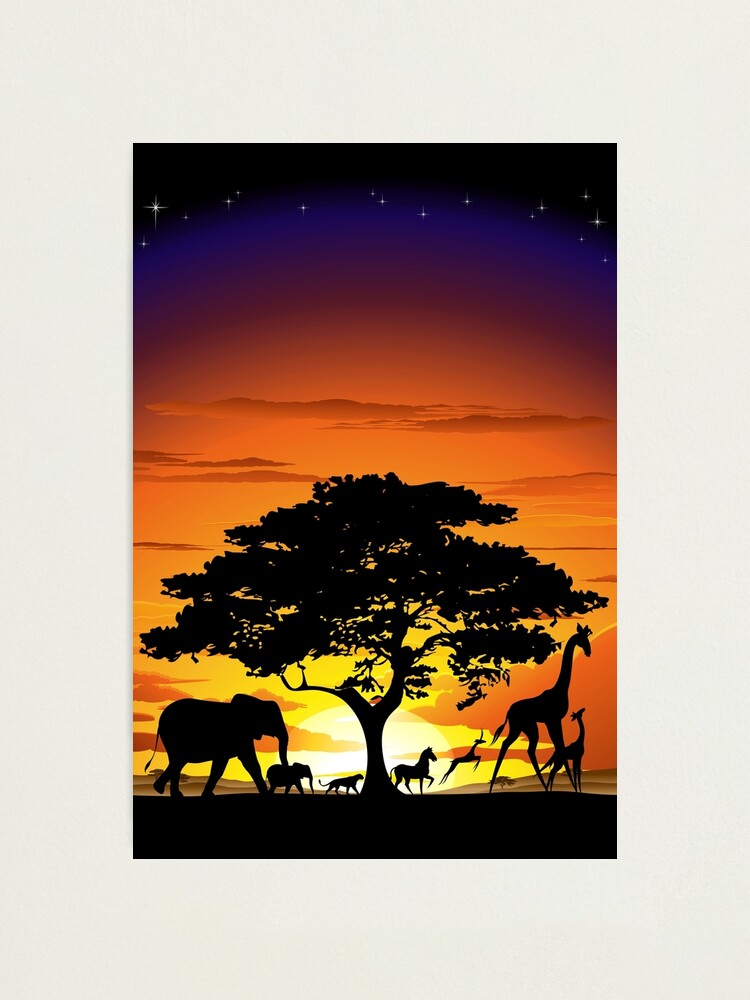This image is an artistic rendering in portrait orientation, framed with a thick, off-white border. It depicts an African landscape at sunset, dominated by the striking silhouette of a large baobab tree in the center. The entirety of the scene, including the tree and animals, is rendered in black, creating a dramatic contrast against the colorful, gradient sky. Surrounding the black tree trunk are a variety of silhouetted animals: on the left, an adult elephant and its calf, and a leopard, while on the right, there's a zebra, a gazelle, and both an adult and a baby giraffe. The ground beneath them is entirely black. The background features a setting sun, its yellow glow transitioning into orange and red clouds. The colors of the sky shift upwards from yellow at the horizon to a darker orange and then blue, eventually fading to black at the top, speckled with stars. Additionally, small brown mountains can be seen on both the left and right sides of the scene, adding depth to this evocative African tableau.